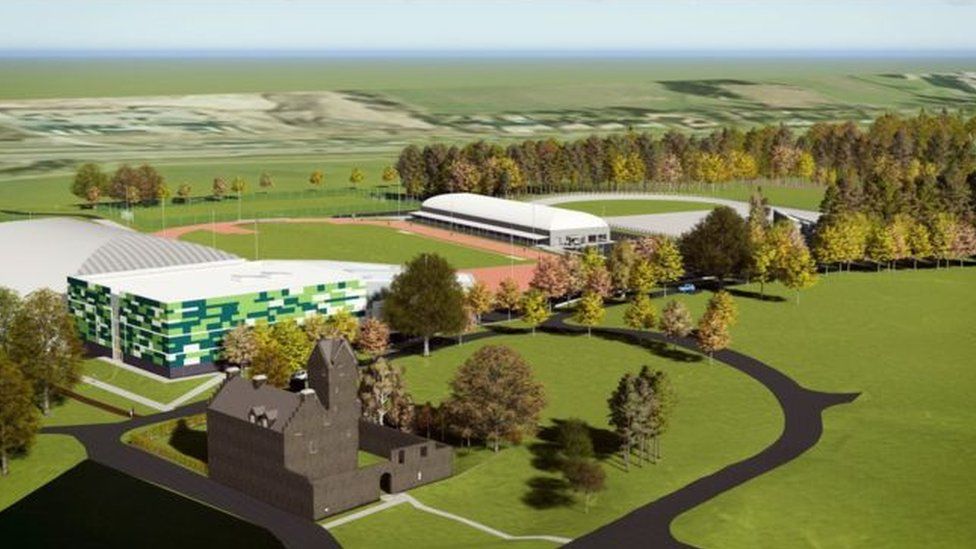This is a photorealistic overhead view of a computer-rendered landscape that appears to be a campus or a sports complex. The scene features a large expanse of green fields interspersed with a few buildings and trees. A striking dark brick building is positioned in the bottom left corner of the image. This building is several stories tall and features a distinct bell tower-like portion, surrounded by a wide driveway and a considerable amount of lawn both inside and outside a fence demarcating the property. Adjacent to this structure is an irregularly checkered contemporary building with a modern design, characterized by a pared-down palette of dark green, light green, and white. There is also a church with a single-material facade, partially enclosing a courtyard. Towards the background, there is a sports field with a track, surrounded by supporting structures on opposite ends. Farther out, more green fields and a lush distribution of trees can be observed, creating a serene and spacious atmosphere, all under a thin slice of light blue sky at the top of the image.